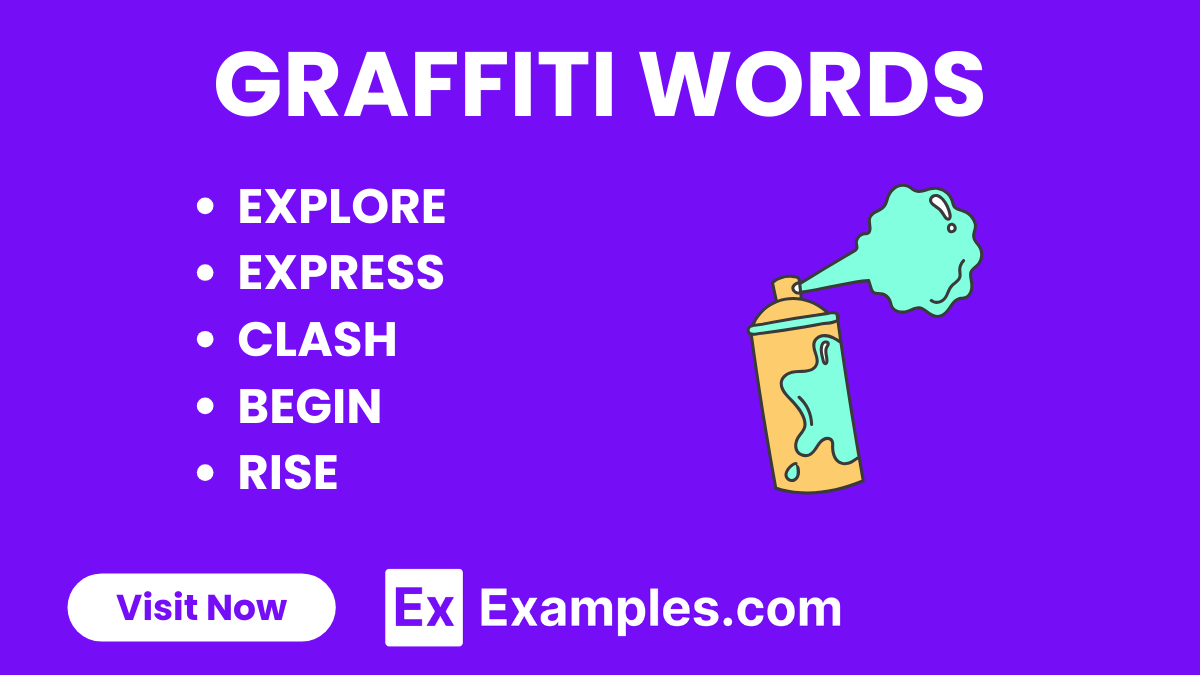The image is a vibrant, color photo of what appears to be a promotional flyer or digital advertisement. Dominating the top is bold, white text proclaiming "Graffiti Words." Beneath this are five key bullet points listed in a vertical arrangement: Explore, Express, Clash, Begin, and Rise, each word individually highlighted. The backdrop features a medium blue to bluish-purple gradient, which offers a contrasting canvas for the vivid elements.

On the right side of the image, an eye-catching spray paint can is depicted. The can itself is a dark gold hue, with blue and orange detailing. It is seen spraying a light mint green paint, which forms a cloud with a white exclamation point inside. Additionally, there is a splash of the same green paint smeared on the side of the can.

In the bottom left corner, within a white oval label, the call-to-action "Visit Now" encourages immediate engagement. On the opposite side, there is a white square featuring the simple, bold letters "EX," next to the URL "examples.com," which presumably directs viewers to a site for graffiti inspiration and ideas. The overall design is dynamic and energetic, with large, capital block letters in white, creating a striking and modern visual appeal.